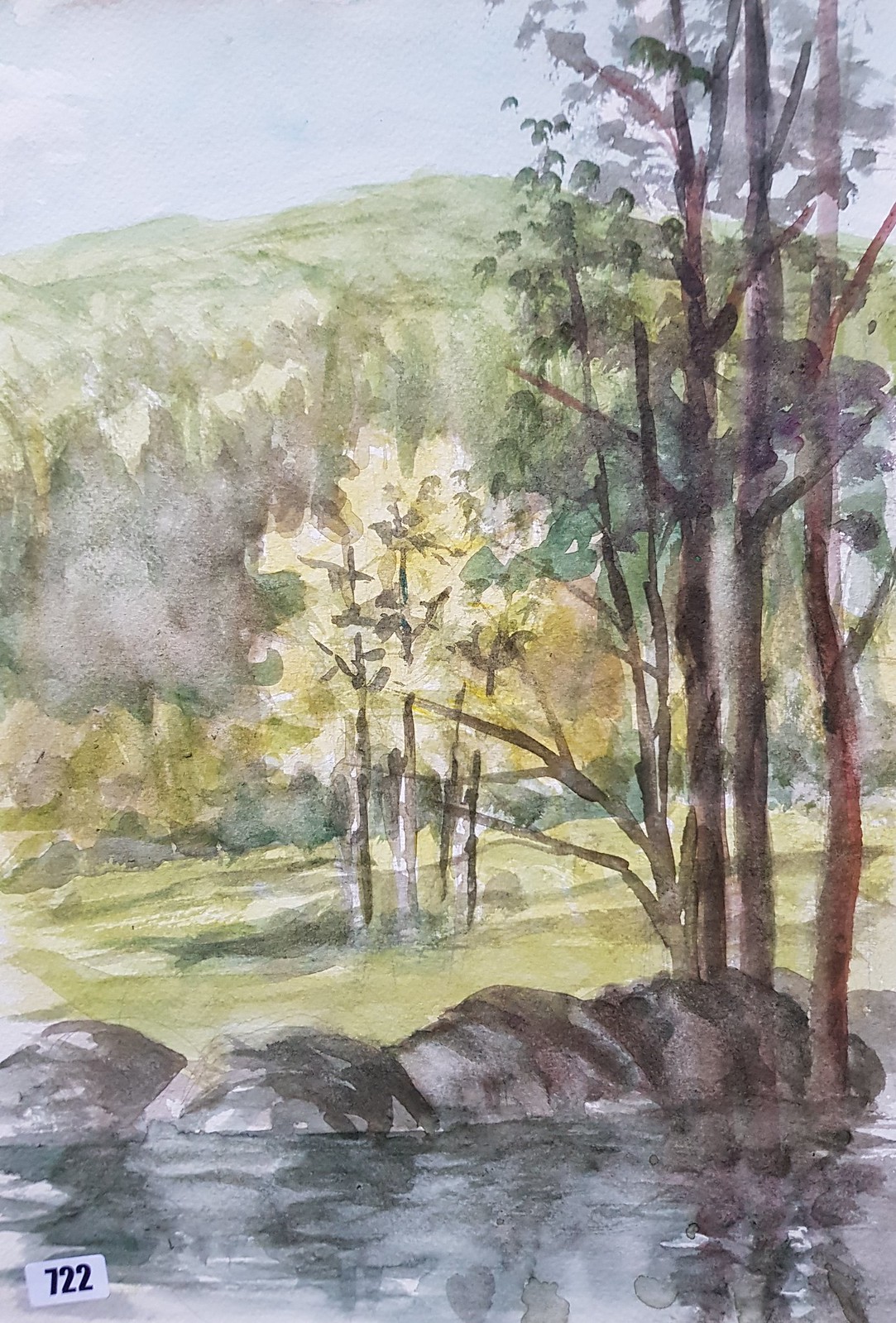This watercolor painting depicts a serene outdoor landscape. In the foreground, a bluish lake, accentuated with greener and darker hues, is bordered by large boulders that transition into lush, green grass. Several bare trees, almost devoid of leaves, grow directly from the water, creating stark reflections in the lake. On the right side, additional trees rise from the rocks, reaching up towards the skyline.

Beyond the lake, a green field dotted with lighter-colored trees extends into the distance. At the center of this field, there's an open clearing highlighted by yellow foliage, creating a contrast with the surrounding greenery. 

Further back, a green mountain range looms, covered in dense, lush vegetation. Above, the sky showcases a mix of purplish and bluish tones, adding to the tranquil yet vibrant atmosphere of the scene.